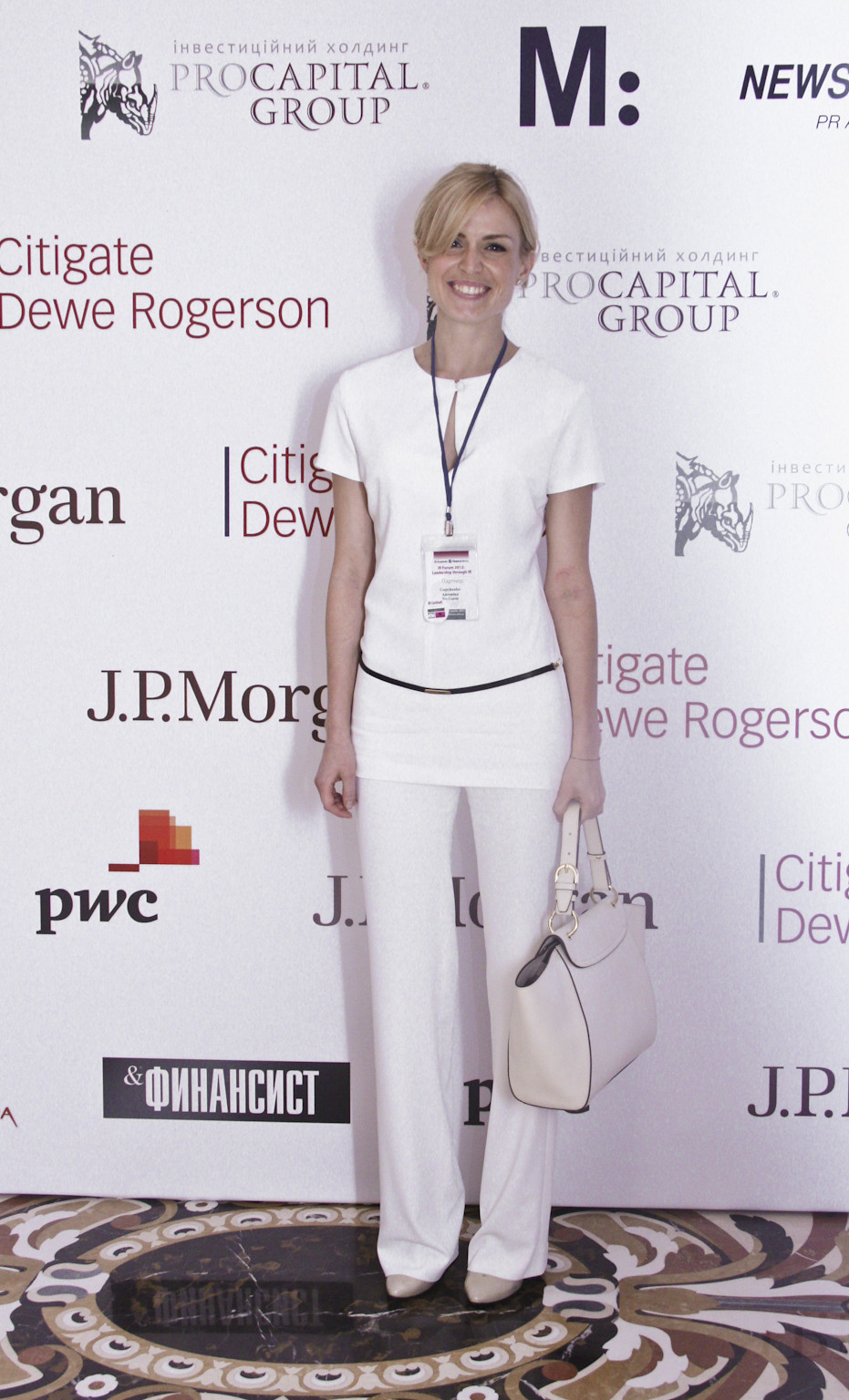A blonde-haired woman with short hair is seen standing upright and smiling at an event. She is dressed in a stylish ensemble consisting of a white shirt tucked into white dress pants, complemented by a thin black belt at her waist. In her hand, she holds a white leather purse, and her feet are adorned in tan dress shoes. Around her neck, she wears a black lanyard with a laminated badge, indicating her credentials for the event.

The woman is positioned in front of a large white banner featuring the logos of several prominent businesses, including Pro Capital Group, CityGate, Rogerson, and J.P. Morgan, among others. The text on the banner is a mix of red, dark brown, and black. The intricate design of the marble floor she stands on features a harmonious blend of brown, white, and black patterns, adding a touch of elegance to the setting.